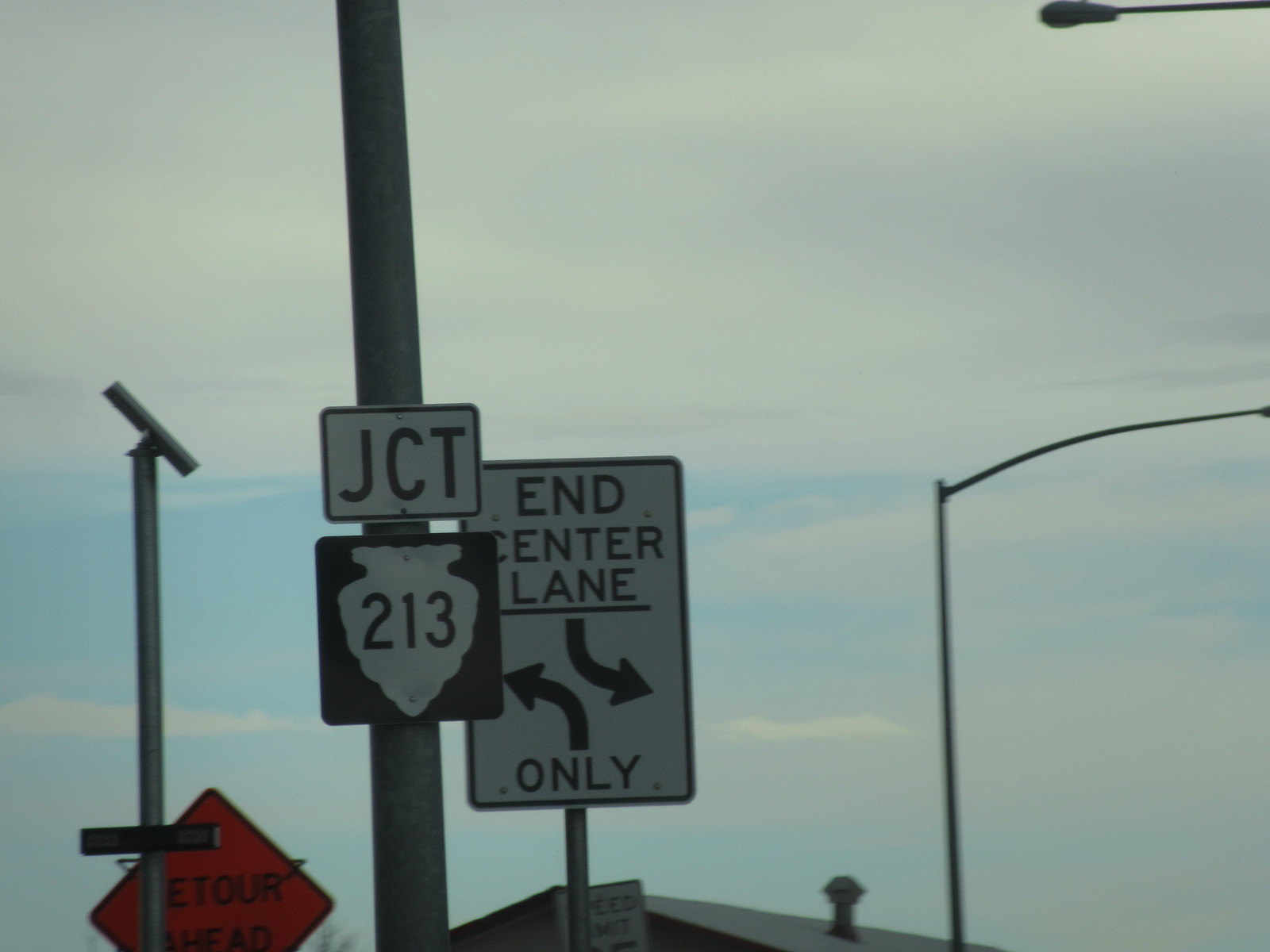In this outdoor photograph, the primary focus is on several street signs situated on a light pole under a partly cloudy sky with patches of blue visible. The upper and lower edges of the image frame the scene without much visible detail apart from the sky, but just beneath the clouds, the faint top of a building or possibly a house can be seen, albeit indistinctly, making it hard to identify. Street lights stand adjacent to the light pole, adding context to the urban setting.

Prominently displayed on the pole is a series of street signs. At the top, a sign reads "JCT 213," which could indicate a junction or a route marker. Below this, an orange diamond-shaped sign warns of a "Detour Ahead," signaling changes or obstructions in traffic flow. At the bottom of the pole, a square sign with the message "End Center Lane" and directional arrows instructs drivers on lane usage. These signs collectively provide a robust direction and caution for those navigating this area.